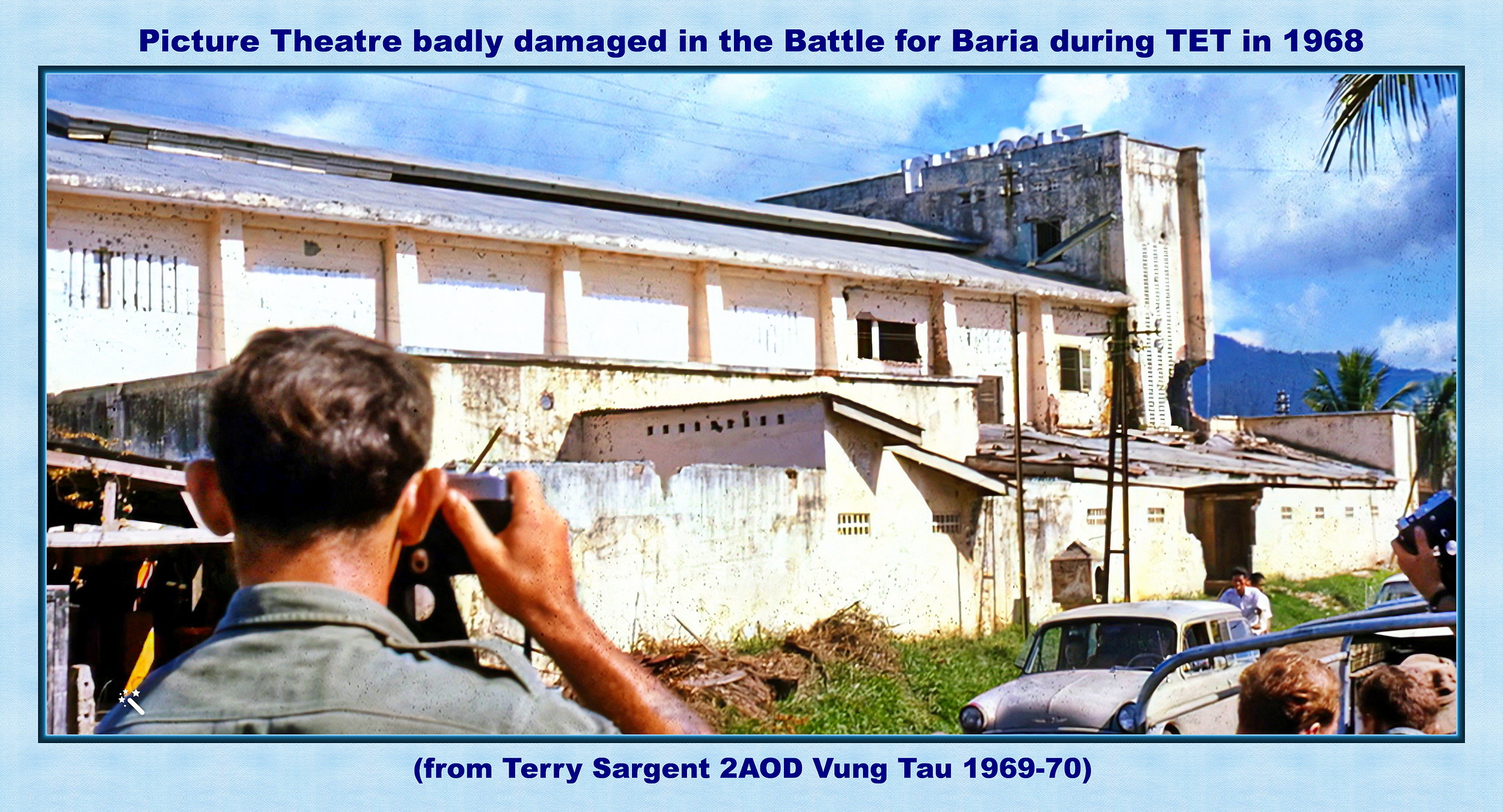The image captures a postcard from the Tet Offensive in 1968, depicting a battle-scarred scene with a tropical backdrop. The two-story building, likely a picture theater, is visibly aged and shows extensive damage with cracks and large holes in its white walls, indicative of mortar strikes. Framing the photo is a teal border, and the background features a light blue sky, partly cloudy. At the top of the image, in prominent dark blue text, it reads: "Picture Theater Badly Damaged in the Battle for Bahria during the Tet Offensive, 1968." Below the photo, in a slightly smaller font, there's an inscription: "(From Terry Sergeant to AOD Vung Tau 1969-70)." Prominent in the foreground is a man capturing a photograph of the ravaged theater using an old camera. Surrounding him are a few older model cars and other individuals, also engrossed in photographing the scene.